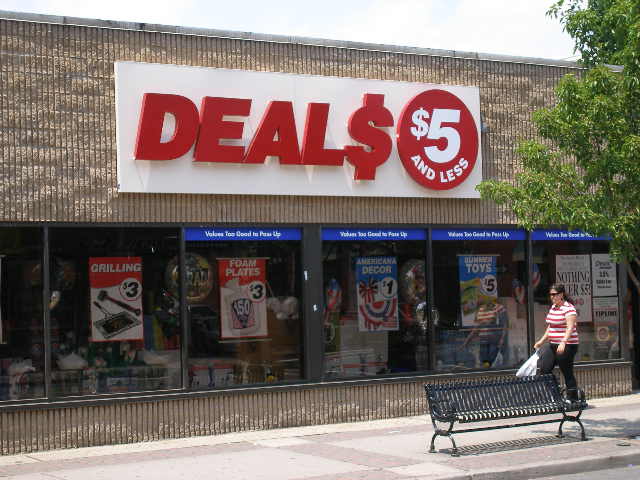In this photograph taken outside a retail store named DEALS, which prominently features a large sign with the word "DEALS" in red, all capital letters, and a dollar sign symbol substituting for the "S," we see an eye-catching storefront. Adjacent to the store name on the right, there's a red circle with white text that announces “$5 and less.” The exterior walls of the store are beige, and the storefront is adorned with five large, tinted glass windows. Each window displays colorful posters advertising various deals: grilling supplies for $3, foam plates for $3, American decor for $1, and toys for $5, among others. 

In front of the store, a woman wearing a red-and-white striped shirt and black pants walks by, carrying a bag in her right hand. She also has sunglasses on. Flanking the scene, a green tree stands on the right, and a black bench sits along the sidewalk. The sky overhead is white and cloudy, casting a diffused light over the entire setting. The overall atmosphere suggests a warm, albeit cloudy day.